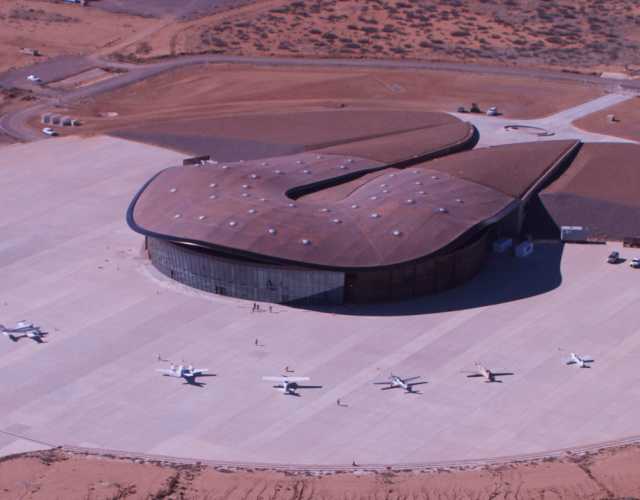The image depicts an overhead, slightly aerial view of a secluded military air force base situated in a desert landscape. The scene is dominated by expansive areas of brown sand and sparse patches of green vegetation, particularly noticeable near the top edge of the frame. A roadway is subtly visible in the background, leading away from the main focus area.

Centrally positioned in the image is a unique, horseshoe-shaped building with a distinct brown, copper-like curved roof that features multiple silver circular fixtures. The structure appears to be one or possibly two stories tall, adorned with glass windows primarily visible on its lower right exterior. A large, light gray tarmac surrounds the building, serving as a parking area for aircraft and vehicles.

Parked on the tarmac are six small aircraft, which seem to be jets or fighter planes, but their exact type remains unclear due to their small size and slight blurriness. A few cars are also seen on the cemented area. In front of the building stand three tiny human figures, indicating some activity at the facility.

Overall, the color palette of the photograph is predominantly brown and gray, reflecting the arid desert environment punctuated with minimal green shrubbery. Shadows cast by the building skew to the right, hinting at the direction of sunlight. The facility, enveloped in a vast, dry terrain, seems like an isolated yet functional air force installation.